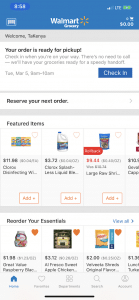The image displays a slightly blurred view of the Walmart Grocery app on a smartphone. Despite the blurriness, it's evident that the main interface showcases a distinctive blue banner at the top, with "Walmart Grocery" written in white text. Next to the text is an icon resembling a star made of orange lines.

At the very top left corner of the screen, you can see the phone's current time, and on the top right, the service provider’s signal strength and battery life indicators are visible. Just beneath the blue banner, there's a personalized greeting that reads "Welcome," followed by a partially indistinguishable name due to the blurriness. 

Directly below the welcome message, the app displays an important notification: "Your order is ready for pickup," accompanied by additional smaller, gray text that is too blurry to decipher. Positioned underneath this notification is a prominent blue "Check-In" button, prompting the user to confirm their arrival for order pickup.

Continuing further down, another option labeled "Reserve your next order" is presented, encouraging users to schedule their future grocery pickups. 

In the subsequent section, the app begins to showcase "Featured Items." This section appears somewhat blurry, but two visible product images hint at some popular items: one resembles a Clorox cleaning product, and another looks like a box of Velveeta mac and cheese, indicating that these might be high-demand items Walmart is promoting.